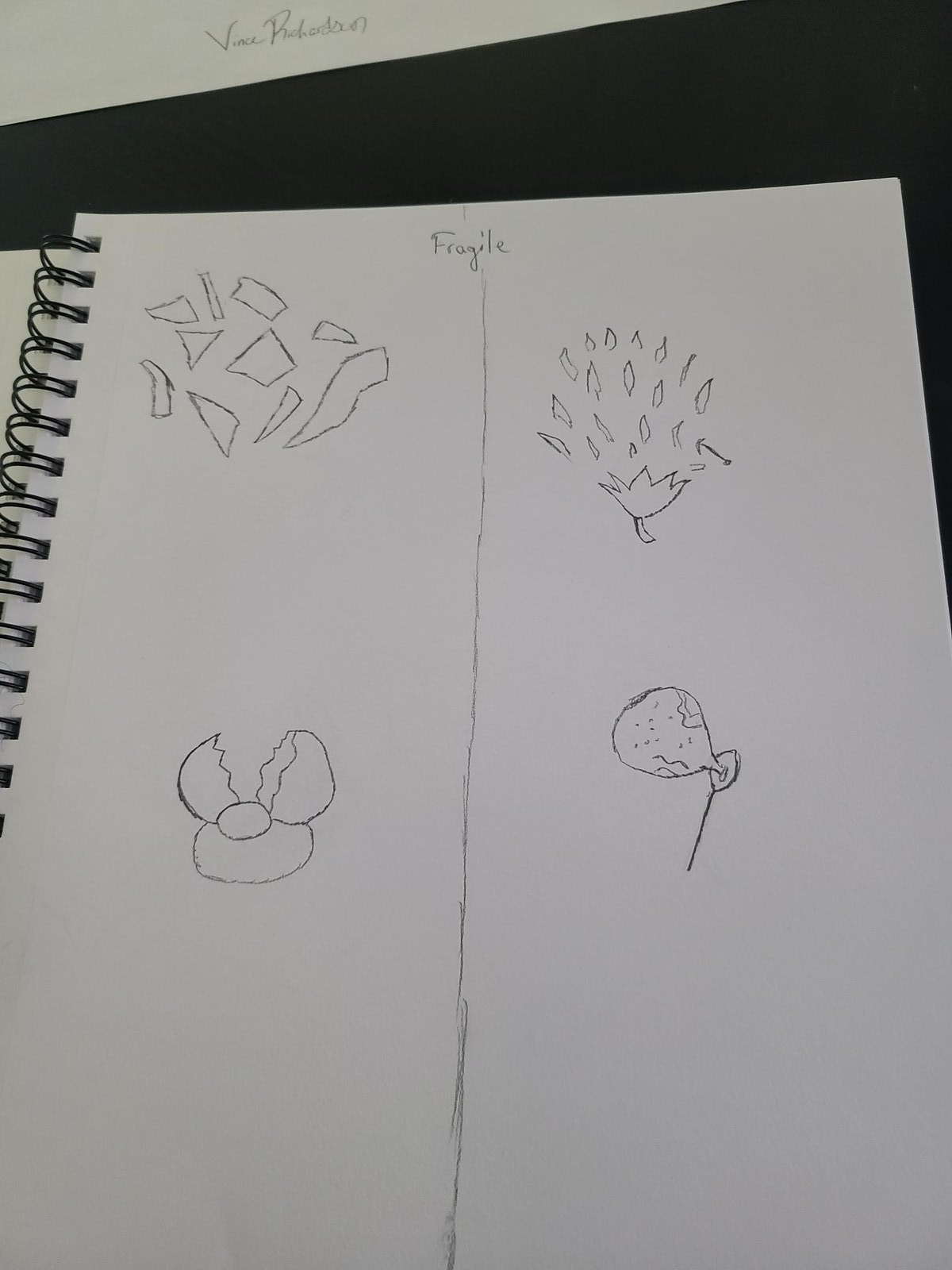The image showcases a sketchbook lying on a black surface. At the top of the photograph, there is a separate white piece of paper signed at the bottom by either Vince Robertson or Vince Richardson. The signature appears to be rendered in pencil, consistent with the medium used in the sketchbook.

The sketchbook, opened to a particular page, features a black spiral binding visible along the left edge, revealing about three-fifths of its length while the rest remains out of the frame. The open page of the sketchbook is white and hosts a series of detailed pencil drawings. A vertical line divides the page into two sections. 

At the top of the page, above the dividing line, the word "FRAGILE" is inscribed. On the left side of the line, there is an intricate depiction of what seems to be shattered glass. To the right of the line, a matchstick with an emerging flame is drawn, though it might also be interpreted as a balloon being punctured by a pin and bursting. Below this, a bubble wand blowing a bubble is illustrated. Adjacent to the bubble wand, crossing back over to the left side of the dividing line, is the drawing of a cracked egg with the yolk spilled out.

All illustrations are meticulously done in pencil, with no use of color, highlighting the artist's skill in shading and line work.